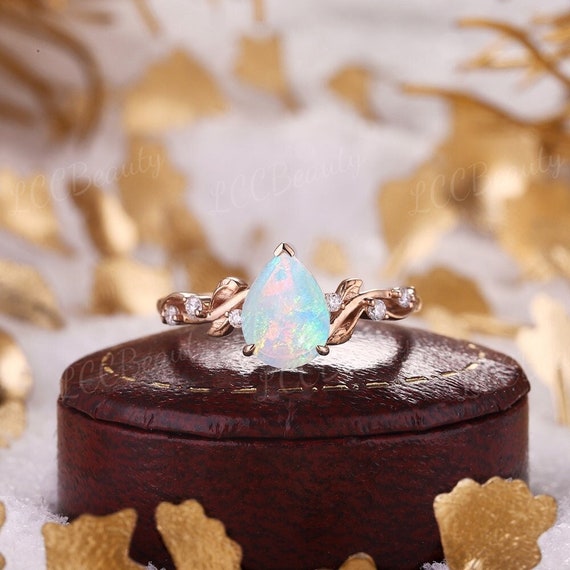This square, color photograph prominently features an opulent gold ring resting atop a circular, dark brown leather case. The centerpiece of the ring is a large, teardrop-shaped opalescent gemstone, shimmering with light blues, pinks, turquoise, and hints of green. Surrounding the central gemstone are at least six small, round white diamonds intricately embedded into a band designed with delicate, gold leaves. The image, likely intended for advertisement, includes a faint, repetitive watermark reading "LCC Beauty," signifying the name of the vendor or company. The background is artistically blurred, emphasizing the ring and its leather base, while faint gold leaves and splotches of white foam encircle the focal point, adding a touch of elegance to the composition.